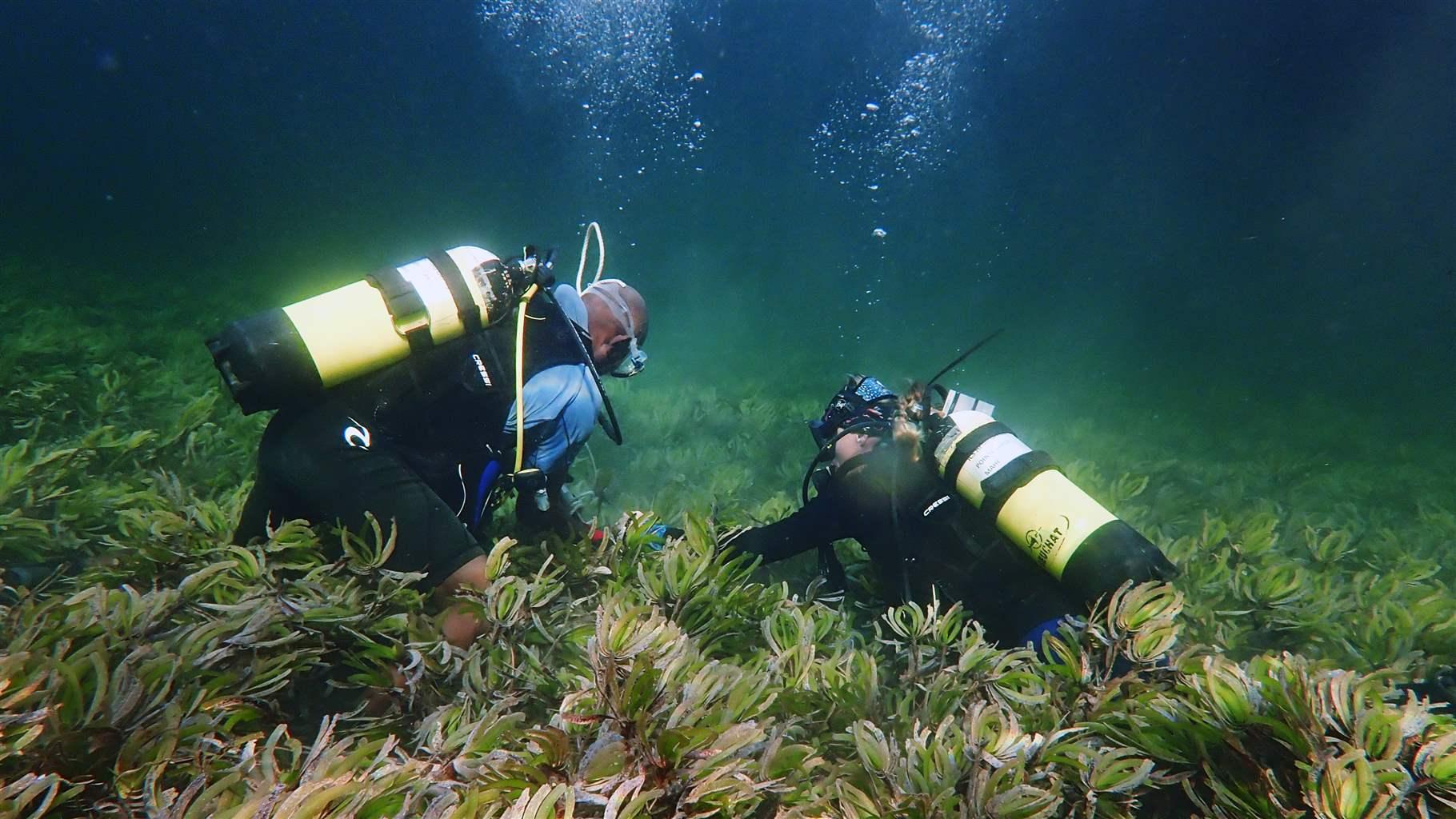In this underwater photograph, two scuba divers are immersed in a murky, dark body of water, surrounded by an abundant growth of green and yellow-green seaweed. Both divers are equipped with yellow and black oxygen tanks, connected to white and yellow hoses, and adorned with necessary scuba gear including vests and goggles. The African-American male diver, wearing a blue and black bodysuit with white symbols, is bent down, seemingly focused on something among the seaweed directly in front of him. The fair-skinned female diver, with blonde hair pulled back in a ponytail beneath her goggles and head strap, is dressed in a black diving suit and appears to be looking intently in the same direction as her partner. Their surroundings are illuminated by sunbeams penetrating the greenish water, which transitions into a darker blue as it recedes upwards. Bubbles rise from their movements, indicating their underwater activity as they work together at the seafloor, possibly in search of something hidden within the aquatic vegetation.